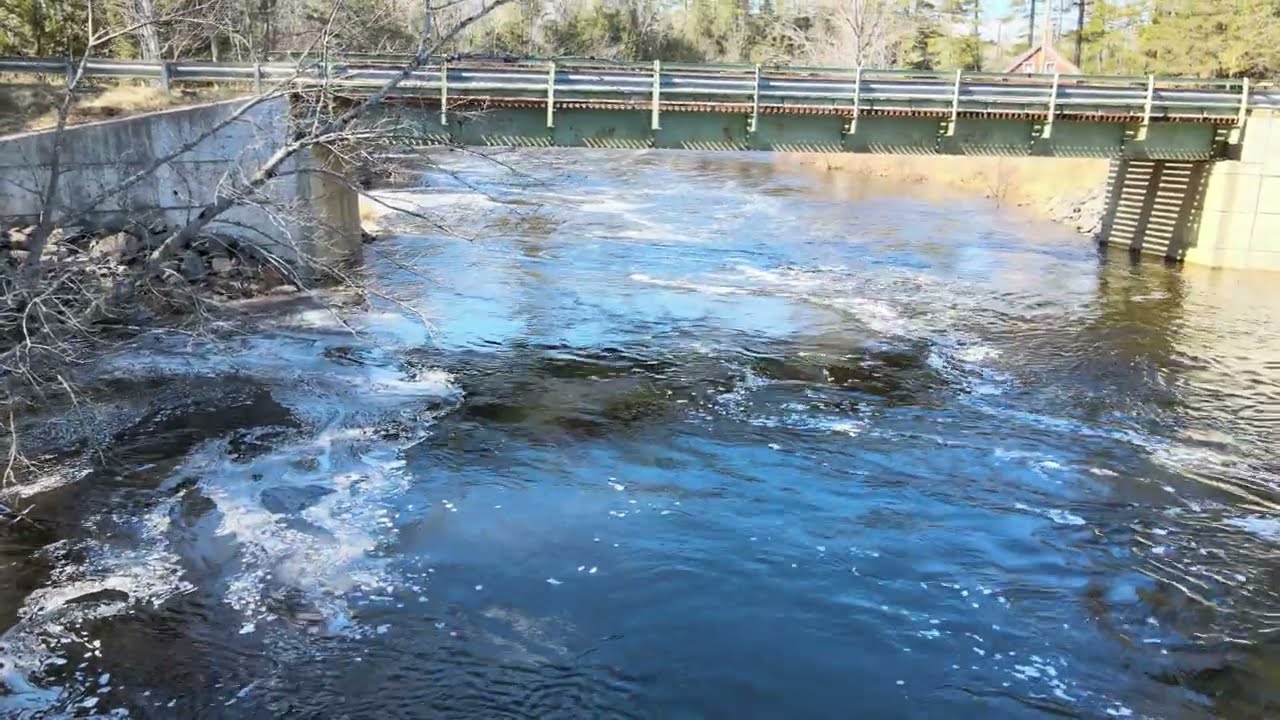The image showcases a wide, shallow, and busy stream seen from a slightly elevated perspective, likely taken from either a drone or a nearby bridge. The stream, characterized by its flowing, frothy, and foamy waters, runs beneath another bridge that spans the top part of the photograph. This bridge is supported by concrete structures on either side and features a green iron beam and a steel guardrail designed to protect vehicles. Shadows cast by the bridge's metal grates are visible along the right side. In the background, amidst a landscape of leafless trees suggesting winter, the roof and upper portion of a house peek through the foliage. The water reveals visible rock formations beneath its surface, indicating both its shallowness and potential danger. Overall, the scene captures a realistic and detailed view of a standard, structurally sound bridge over a regional stream, framed by seasonal vegetation and a hint of rural habitation.